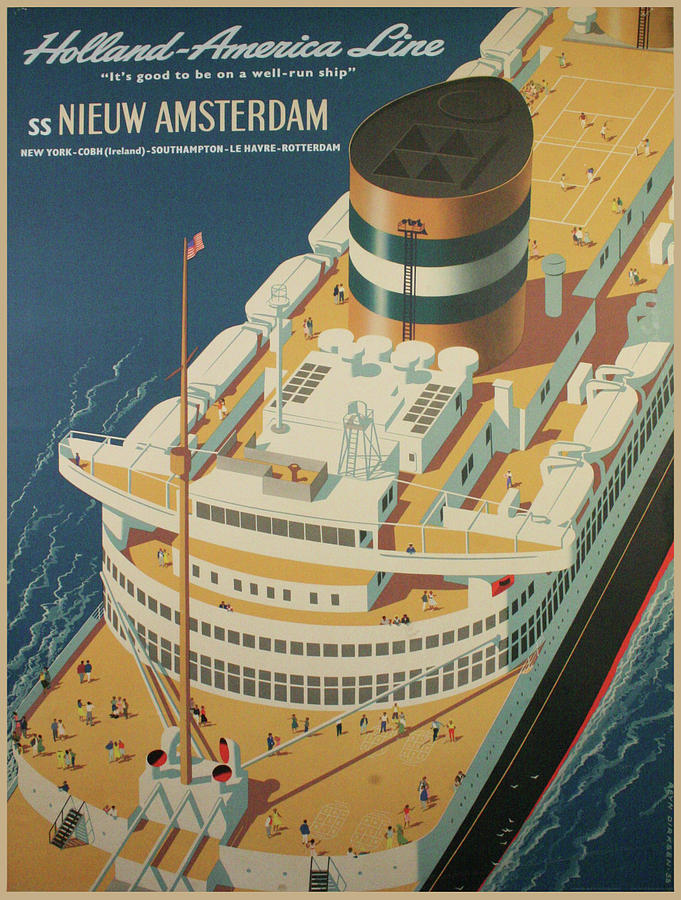The advertisement poster for the Holland America Line features a 1920s art style with a light brown border. Dominating the image is a colorful, cartoon-like depiction of the SS Nieuw Amsterdam cruise ship, viewed from the top down. The title "Holland America Line" is elegantly written in light blue cursive at the top left, just above the quote "It's good to be on a well-run ship." Beneath the quote, the ship's name "SS Nieuw Amsterdam" (with "Nieuw" spelled N-I-E-U-W) is prominently displayed in light blue and light brown font. Below the ship’s name, fine white print lists its travel route: New York-Copenhagen, Ireland-Southampton-Le Havre-Rotterdam.

The ship's decks are depicted in yellow with black sides featuring a red stripe at the waterline. The smokestack is decorated with yellow, blue, and white stripes. Visible are white lifeboats lined up, a tall flagpole flying a small American flag, and several tiny, indistinct figures representing passengers along the railings and on the decks. The scene captures the daily activities of these miniature figures, appearing like tiny ants in various colors such as yellow, red, blue, and green, adding a sense of bustling life to the ship.

The detailed artwork includes a big smokestack, stairways, and a small tower structure where one might imagine a lookout. The surrounding blue water features subtle white lines indicating waves, enhancing the maritime ambiance of this charmingly nostalgic advertisement.